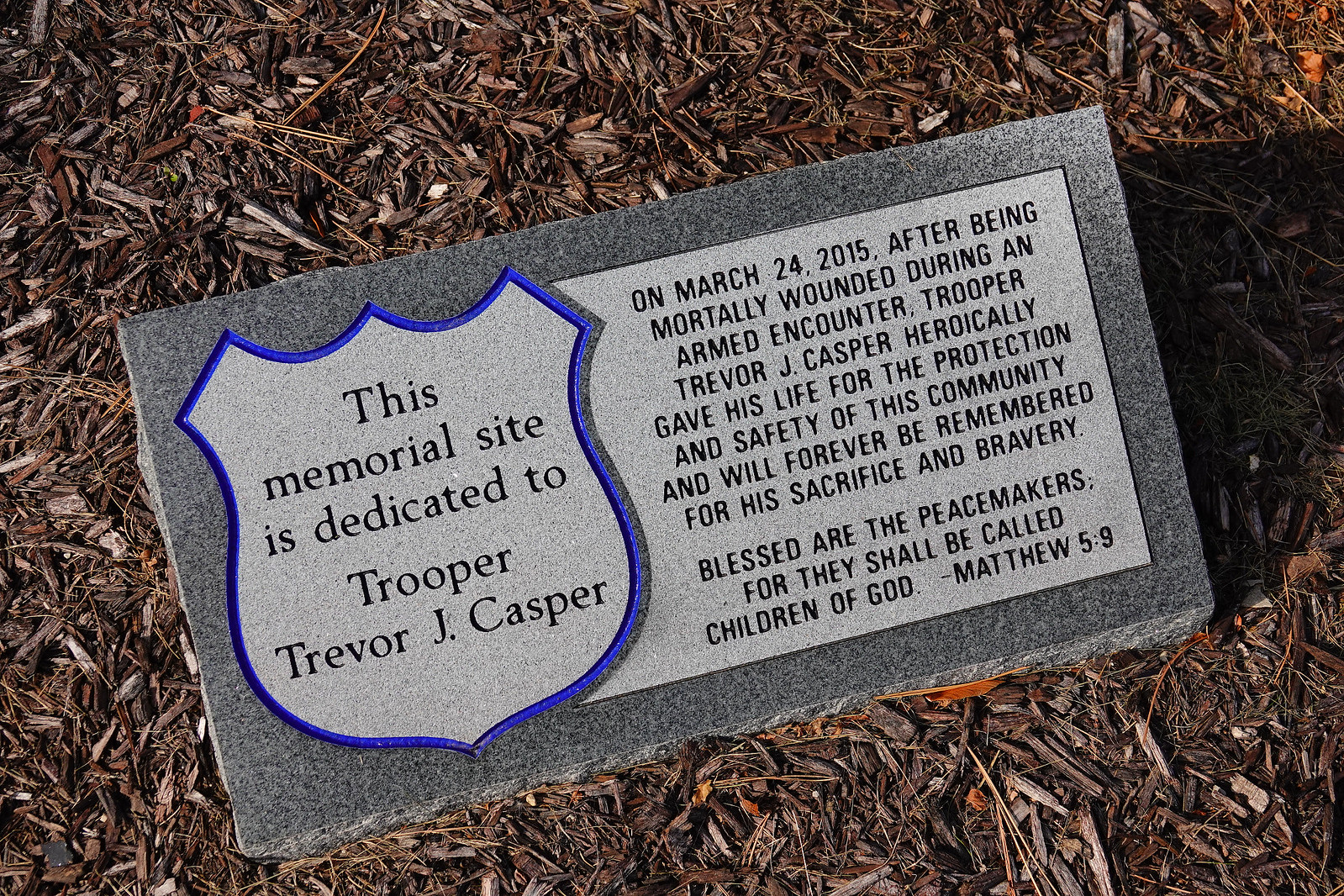The image depicts a gray granite memorial plaque, slightly angled upwards, embedded in a ground covered with dried grass, sticks, bark, and mulch, resembling a grave site. The focal point of the memorial is a blue-bordered police badge on the left side, which reads, "This memorial site is dedicated to Trooper Trevor J. Casper." To the right of the badge, an inscription in black writing states, "On March 24, 2015, after being mortally wounded during an armed encounter, Trooper Trevor J. Casper heroically gave his life for the protection and safety of this community and will forever be remembered for his sacrifice and bravery. Blessed are the peacemakers, for they shall be called children of God. Matthew 5:9." The surrounding background consists predominantly of brown tones, emphasizing the somber nature of this tribute.